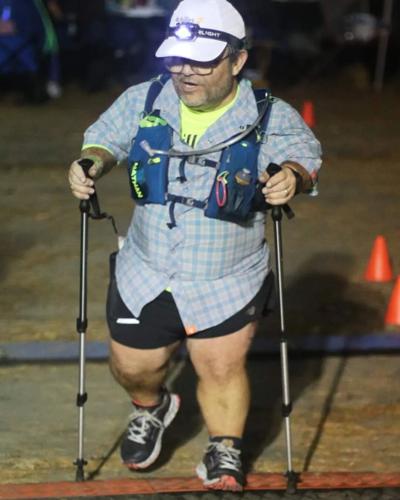This is a detailed, real-life color photograph taken predominantly outdoors, likely during a nighttime rally or marathon for disabled individuals. The focus is on a short-statured man, approximately in his late 40s or early 50s, who is walking with the aid of two telescoping crutches. He is dressed in practical hiking gear which includes a white baseball cap with an attached headlight that is switched on. His outfit consists of a blue-and-white plaid button-down shirt over a yellow T-shirt, accompanied by a blue utility vest with multiple pockets and some unreadable yellow text. The man also sports tight black shorts, black sneakers with white laces, and glasses. His determined expression is accentuated by his sturdy build. The scene is set against a backdrop of a darkened sky with orange construction cones and blurred markers on what appears to be a pavement or road, suggesting the area might be sectioned off for the event.